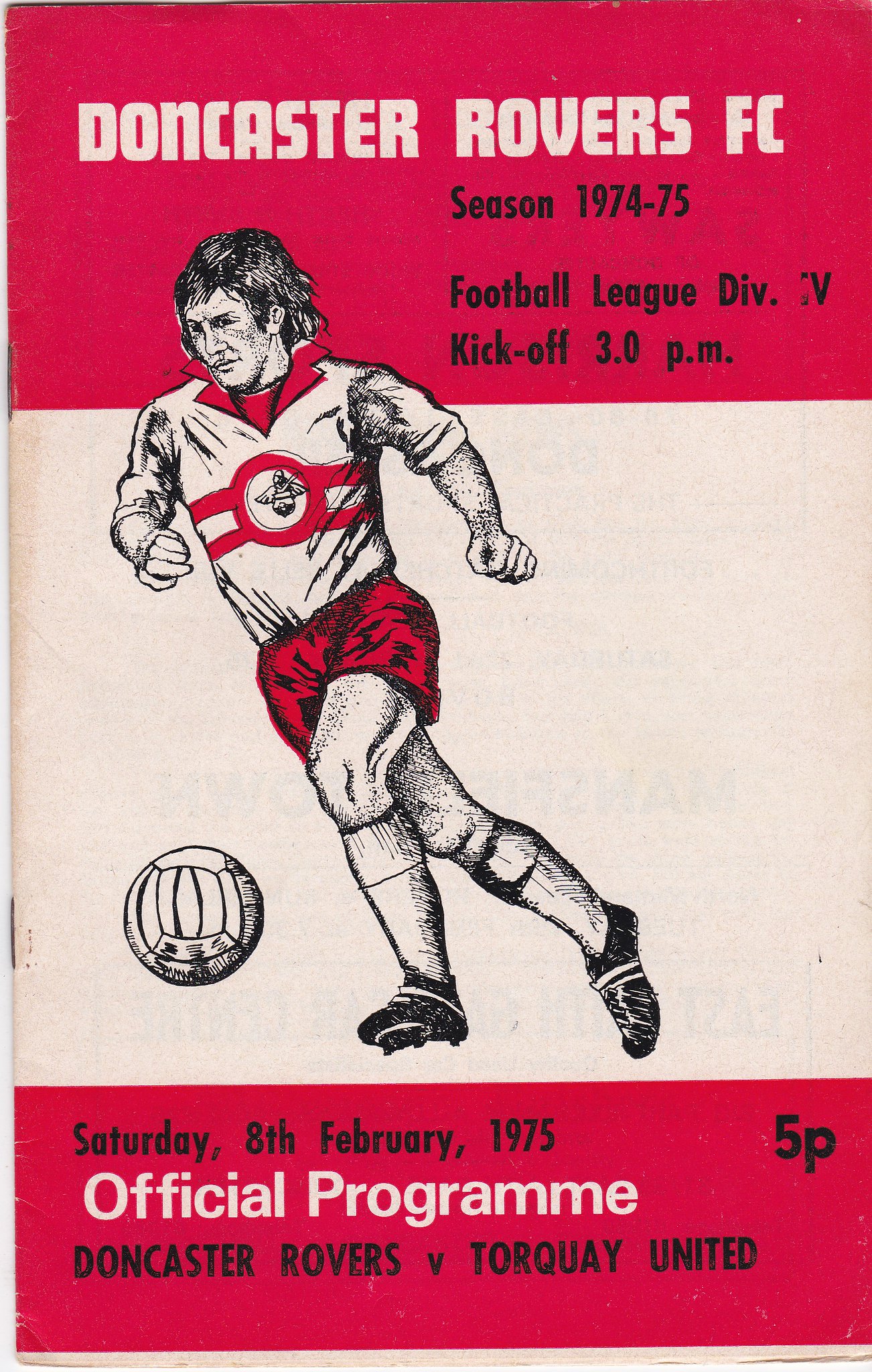The cover of the Doncaster Rovers FC official program is a vertical rectangular image, prominently featuring wide red bands at both the top and bottom, with white and black lettering. The top red band displays "Doncaster Rovers FC," with the text "Season 1974-75, Football League Division IV, kickoff at 3.00 p.m." in black just below. The center of the cover has a white background that showcases an illustrated soccer player in action, dressed in the team’s uniform of red shorts and a white shirt accented with red bars and a red collar. The player is depicted mid-run, poised to kick a soccer ball. The bottom red band contains further details: "Saturday, 8th February 1975, Official Program Doncaster Rovers versus Torquay United, 5P." The illustrated character and overall design give the program a lively, animated feel, with some tan colors evident and staples along the side indicating it’s part of a multi-page booklet.